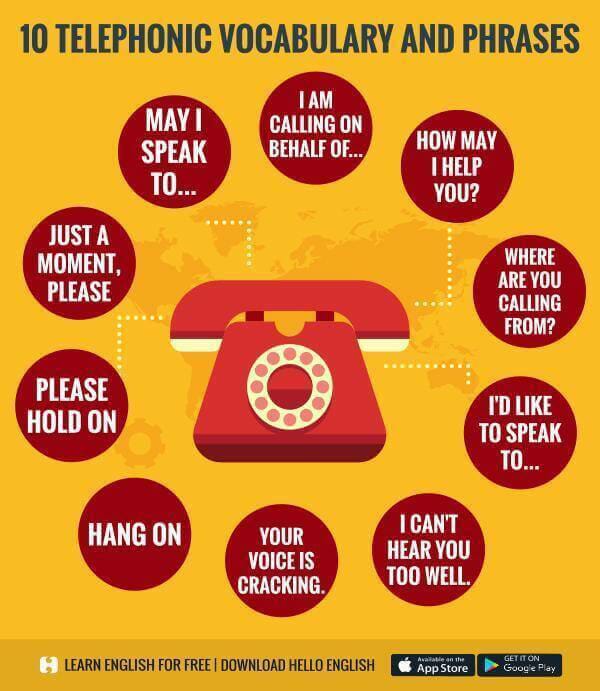This vibrant infographic poster, set against a yellow background featuring a subtle world map, prominently displays the title "10 Telephonic Vocabulary and Phrases" in a dark blue font at the top. Central to the poster is a cartoonish, light red rotary phone, symbolizing traditional telephonic communication. Surrounding this phone are ten commonly used phrases in telephonic conversations, each encapsulated in dark reddish circles with white text. The phrases, arranged in a clockwise manner, include:

1. I am calling on behalf of
2. How may I help you?
3. Where are you calling from?
4. I'd like to speak to
5. I can't hear you too well
6. Your voice is cracking
7. Hang on
8. Please hold on
9. Just a moment please
10. May I speak to

At the base of the poster, a call-to-action reads "Learn English for free, download Hello English," accompanied by logos for the Apple App Store and Google Play Store, encouraging viewers to further their language skills.